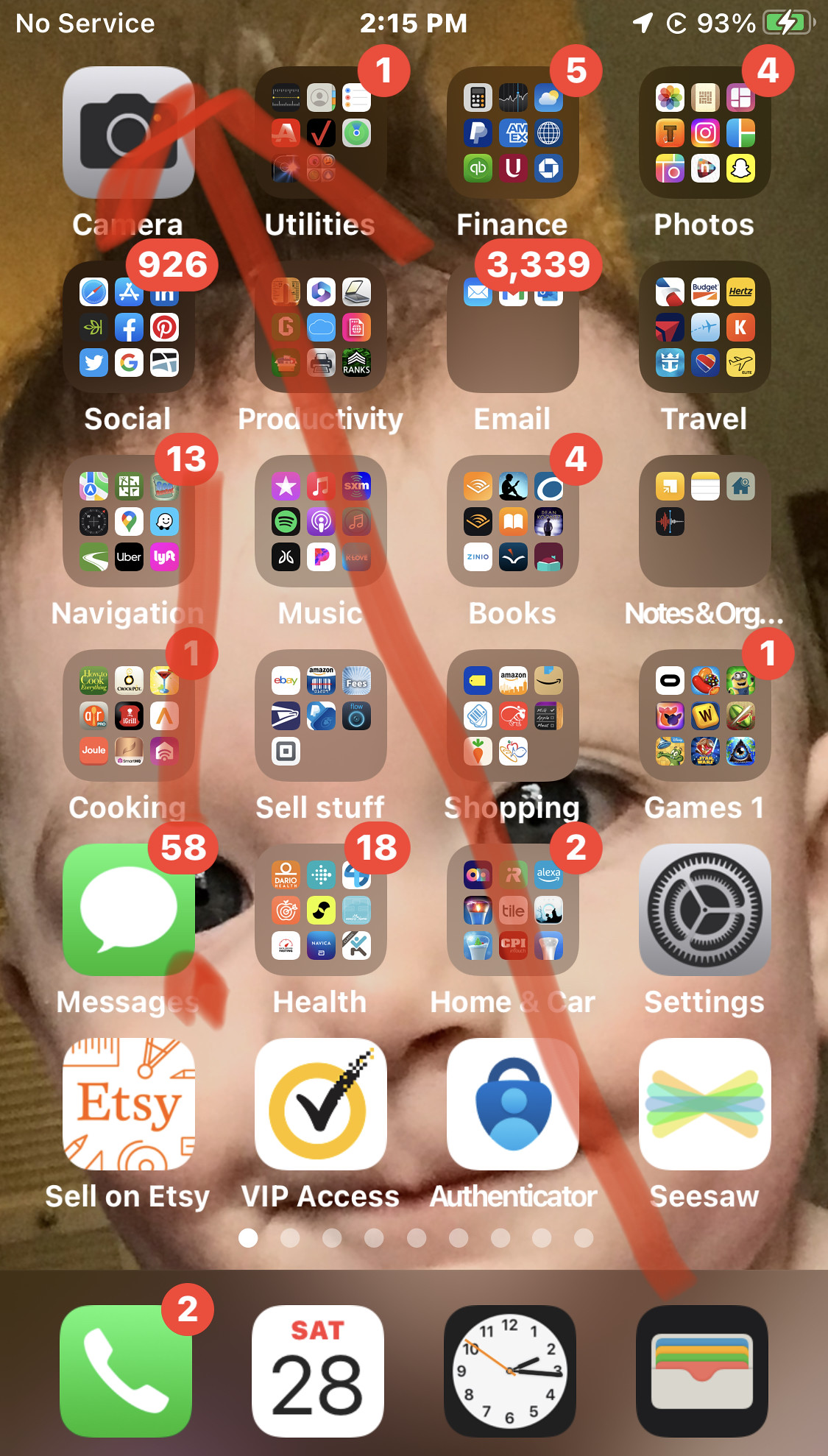Screenshot of an Apple iPhone Interface: The screenshot depicts an iPhone interface, identifiable by the layout and design of the icons which appear slightly bulkier compared to Android devices. The status bar at the top displays “No Service” on the left, “2:15 PM” in the center, and a battery icon at 93% on the right. Additionally, there is a small arrow symbol, suggesting active notifications, near the battery indicator, and all of these elements are displayed in white.

On the home screen, the top-left icon is a camera. Adjacent to it are folders labeled “Utilities,” “Finance,” and “Photos.” The second row contains folders for “Social,” “Productivity,” “Email,” and “Travel.” The third row includes “Navigation,” “Music,” “Books,” and “Notes & Organization” (with the latter truncated as “Notes and org…”). The fourth row displays folders for “Cooking,” “Cell,” “Stuff,” “Shopping,” and “Games.” Below these, individual apps are arranged: “Messages,” “Health,” “Home” and “Car Settings.”

The final row includes apps named “Cell on Etsy,” “VIP Access,” “Authenticator,” and “Seesaw.” At the bottom of the screen sits the dock, featuring a green “Phone” app square with a red notification badge indicating two missed calls or messages. To the right of the Phone app, a calendar icon displays “Saturday 28.” Next to it, there is an icon resembling a watch face, followed by what appears to be a Photos app icon.

The wallpaper in the background is an adorable image of a baby’s face, adding a personal touch to the device interface.